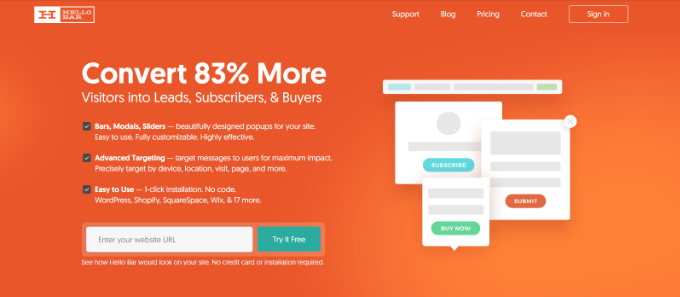This image showcases an advertisement for a marketing tool called "Hello Bar." The ad promotes a service designed to convert website visitors into leads, subscribers, and buyers with an 83% higher conversion rate. It emphasizes advanced targeting features that are easy to use, catering to companies aiming to enhance their marketing strategies through data-driven methods. The visual presentation includes an orange background with chat bubbles and a sign-up screen, reflecting a standard user interface commonly seen on contemporary websites.